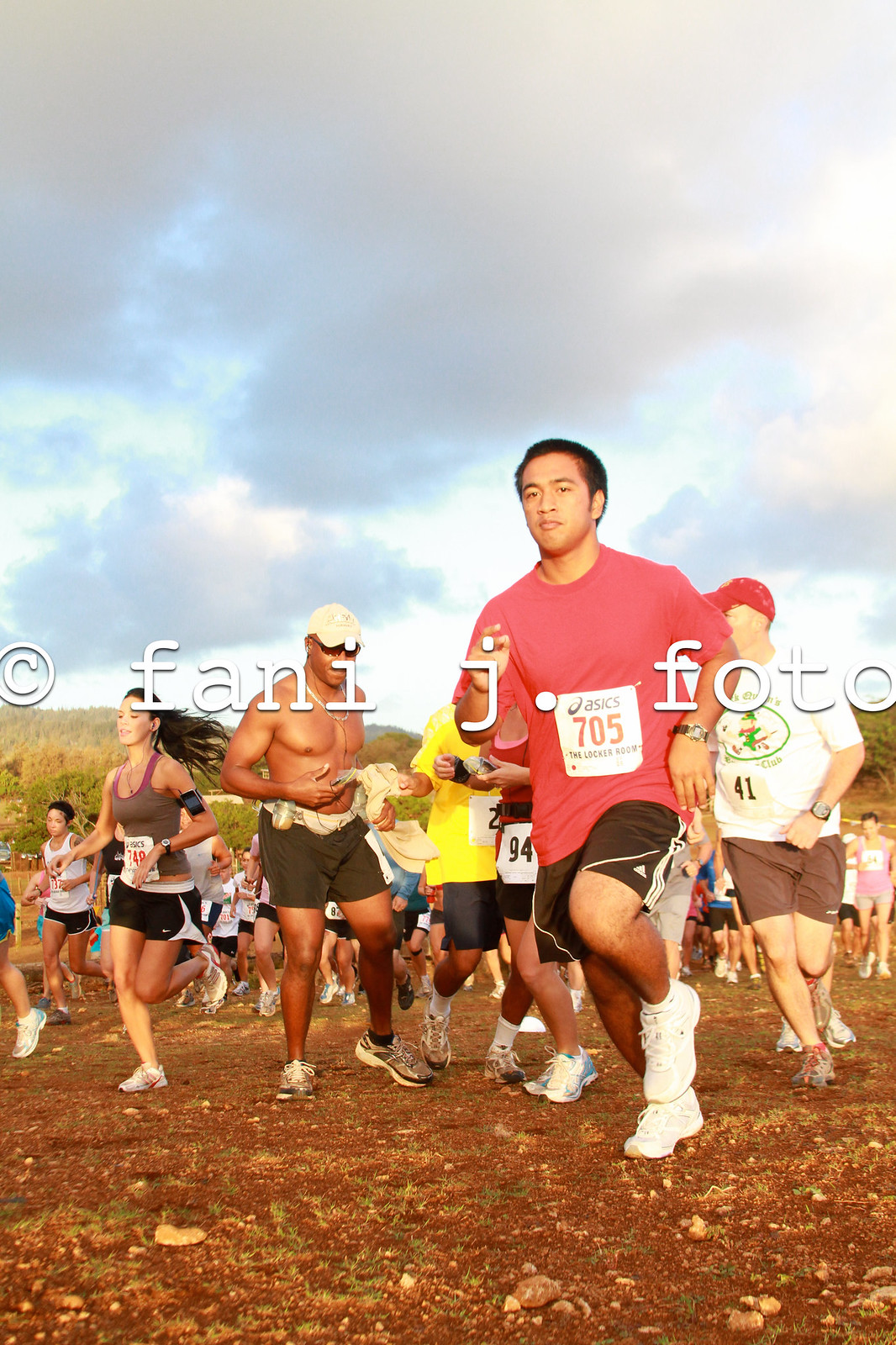In this photograph, taken outdoors at a race event, the scene is set under a predominantly cloudy sky with glimpses of light blue peeking through. The landscape features grassy hills against which a multitude of runners are captured in various stages of movement along a dirt path. The prominent watermark on the image reads "© Fanny J. Photo."

In the foreground, a man of color wearing a red T-shirt numbered 705, black shorts, and white running shoes stands out. Beside him, a shirtless man sporting dark greenish-gray shorts and holding a brown hat appears to be taking a momentary break, directly engaging with the camera. To their left, a woman with long, dark hair pulled back by the breeze dons a gray tank top with purple straps, black shorts, and white running shoes while continuing her run. Further to the right, another distinguishable runner wears a white T-shirt, brown shorts, and a red baseball cap. All participants are diverse in age and style, contributing to the dynamic energy of the event. The background and the runners' varied details, including numbered bibs and distinctive attire, encapsulate the spirit and diversity of this lively race.